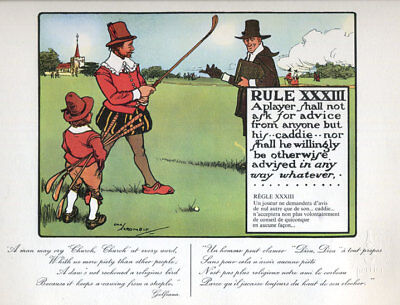This detailed illustration, evocative of early colonial times, depicts a scene of individuals engaging in a round of golf on a lush green course beneath a clear blue sky. The characters are attired in historical clothing, with one figure resembling a pilgrim, donning a black hat and suit. Accompanying him are others dressed in vibrant red coats with brown hats, and wearing voluminous pants puffed at the hips. One noticeable figure, potentially an official or judge, dressed in traditional pilgrim attire, stands out with red shoes and a unique, period-specific golf club. Adjacent to him, a young boy, serving as a caddy, holds additional clubs. The backdrop features a building with a red roof and surrounding trees. Prominently displayed within a text box on the right is Rule Number 33, articulated in Roman numerals, admonishing players that they "shall not ask for advice from anyone but their caddy." Beneath the illustration and framing it generously are a couple of cursive-written paragraphs, albeit too small and faded to decipher, likely containing further insights or directives on the rules of golf.